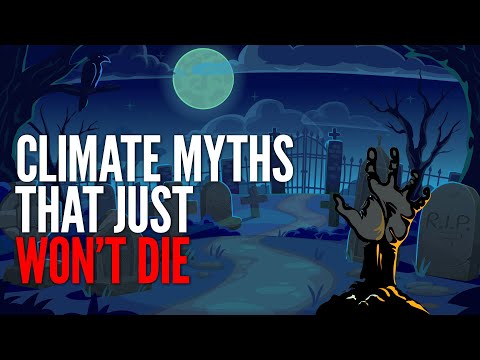The image is a detailed cartoon art piece depicting a nighttime cemetery scene, which appears to be a screenshot from an animated video. The central focus of the image is the title "Climate Myths that Just Won't Die," written in capital letters, with the words "won't die" in red and the rest in white. The background features a large, silvery bluish-green full moon partially obscured by clouds, situated slightly left of center at the top. The foreground is dominated by a graveyard with a prominent hand emerging from the ground on the right, starkly illustrated in black and gray, with the wrist visible above a small black mound of dirt. Surrounding the hand are several gravestones, including one prominently marked "R.I.P." and others featuring cross shapes. A metal fence and gates enclose the graveyard, and a dark bird, resembling a crow or raven, perches on a tree branch on the left side. The image also includes a mix of black and blue backgrounds, adding to the eerie, symmetrical nighttime ambiance.